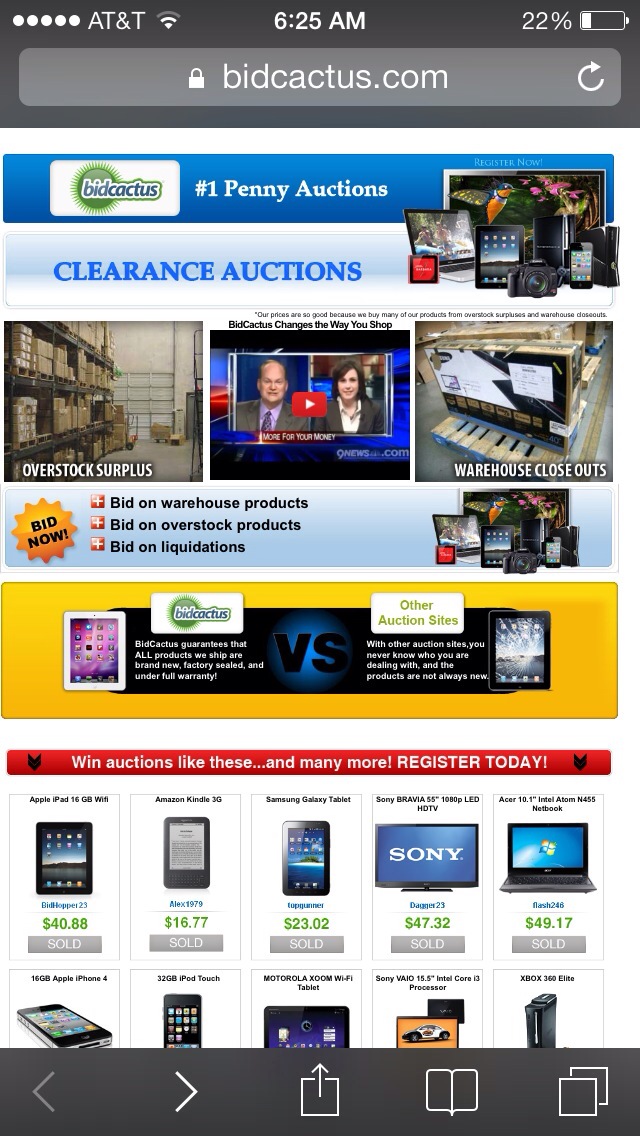The image is a detailed screenshot from the front display of a smartphone, specifically an iPhone, with AT&T service and connected to Wi-Fi, symbolized by a small triangular icon. The time displayed is 6:25 AM, and the battery is at 22%. At the top of the phone screen, there's a search bar showing the URL "BidCactus.com," indicating the user is on a penny auction website named BidCactus. 

Below the search bar, a blue header with the BidCactus logo is prominent, featuring a green circle with spines, and the text "BidCactus" in blue next to it. The banner also claims to be the "Number One Penny Auctions" site. A section labeled "Clearance Auctions" is visible, showcasing various items available for bidding, such as iPads, smartphones, laptops, and a television priced at $47 and $49 respectively. Additionally, there are images suggesting overstock surplus items and what appears to be a YouTube video about the auctions. A yellow badge with red text says "Bid Now," and bullet points below highlight options to bid on warehouse products, overstock products, and liquidations. The bottom section features the BidCactus logo again, comparative text about other auction sites, and a "Versus" notation, though the differentiating details are too small to read. The phone's web interface controls can be seen at the bottom of the screen.